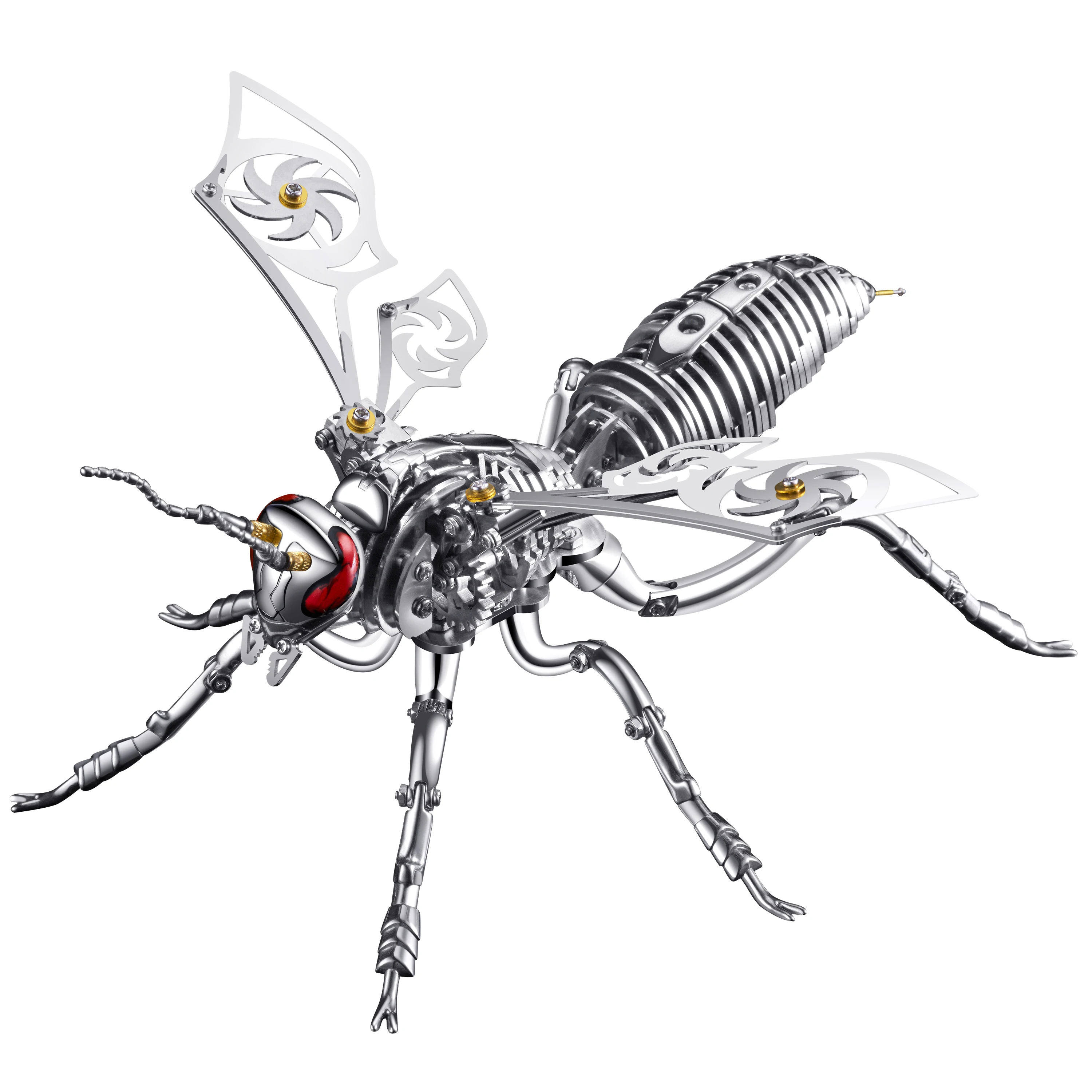The image features a highly detailed, intricately designed metallic insect resembling a wasp or an ant, set against a plain white background. The insect's mechanical wings, which appear to contain elements similar to Chinese throwing stars or blades, suggest potential movement powered by visible gears. The body is composed of solid silvery metal, with the abdomen resembling a spring, culminating in a sharp stinger. The insect's six articulating legs, fastened with screw-like joints, end in pointed feet, adding to its lifelike appearance. Prominent red eyes stand out on its head, along with antennae and pinchers, enhancing its menacing look. The image appears to be a highly detailed drawing, possibly for a game or a comic, with the insect oriented diagonally from the bottom left to the top right of the frame. The precise craftsmanship and complex design elements hint at it being a standalone piece of intricate mechanical artwork.